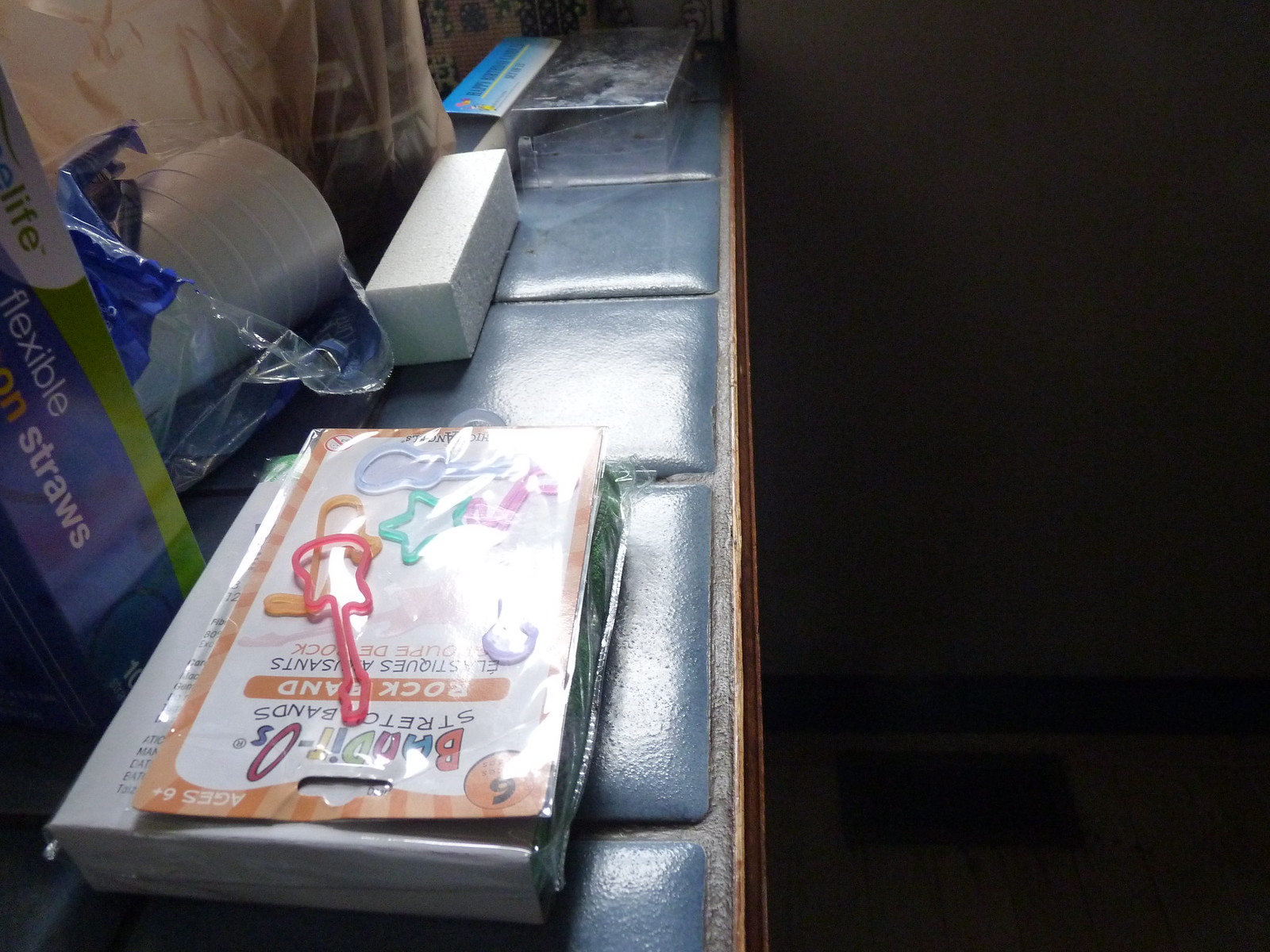A picture of a blue textured countertop situated in a dimly lit room, with the light fading towards the right. The darkened right side reveals a faint wall featuring darker wood paneling and a wooden floor with visible beams. A small welcome mat is situated on the floor. The countertop itself is distinctly textured with a plastic-like surface and brown edges. Various objects are scattered across it, including a white plastic container in the foreground holding some towels or sheets. Placed on top are colorful gel stickers shaped like guitars in red, green, blue, and purple, encased in plastic packaging and mounted on cardboard with an orange border. A box of blue and green plastic straws, a cylindrical roll of fabric wrapped in blue and white paper, orangish fabric draping around, and an empty container sit at the far end of the countertop.